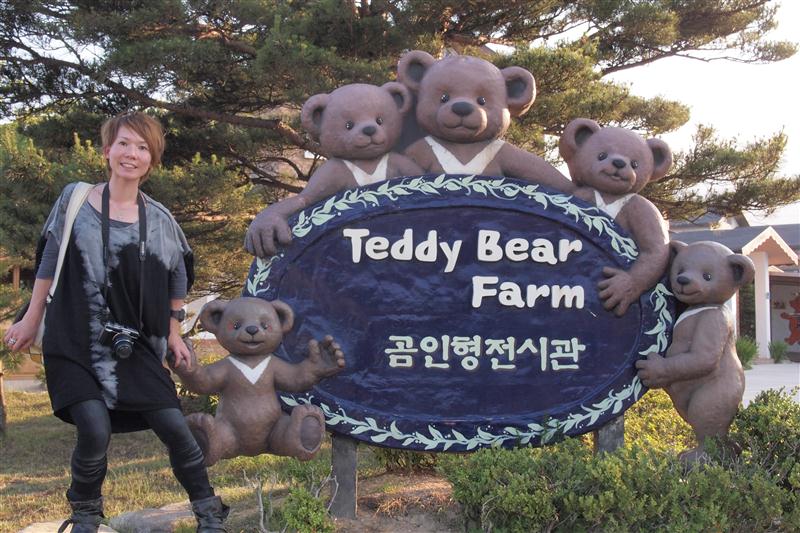The image is a realistic outdoor photograph taken during the daytime, framed in a horizontal rectangle. In the background, the sky appears light gray and bright. The center and lower portions of the background feature tall green bushes and a prominent tall pine tree. To the back right, there's a partially visible building with white pillars and a gray tiled roof.

In the foreground, there's a dirt path with patches of grass on the left and short green bushes on the right. Central to the scene is a large, oval-shaped blue sign with white lettering that reads "Teddy Bear Farm" along with Asian characters, possibly Japanese, beneath it. The sign is adorned with a light green flowery trim and five brown teddy bear statues, each with a white V-shaped mark on their chest, positioned around the sign.

Standing to the left of the sign is an Asian woman with light skin and reddish hair, dressed in a black and gray outfit with black leggings. She has a camera hanging around her neck and a white purse. The woman, who appears to be in her 20s or 30s, is smiling at the camera while holding the outstretched hand of one of the bear statues. The scene is set against a backdrop of greenery and an indistinct building, creating a charming and inviting atmosphere.